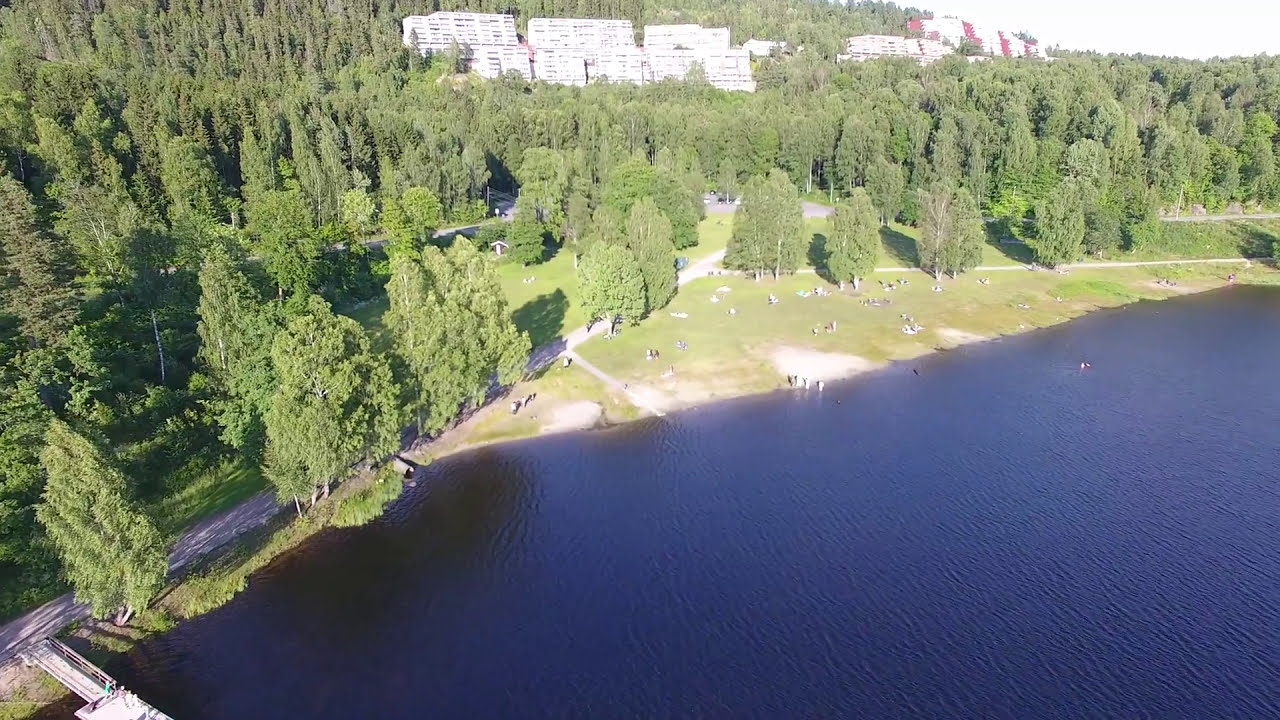Looking down from an overhead view, this striking summertime image captures a navy blue lake with light ripples on its surface. The body of water stretches from the bottom right up to nearly halfway through the picture. Surrounding the lake is an expansive, grassy area with varying shades of green and yellow, dotted with people relaxing on patches of grass and dirt. There is no sandy beach, but the green fields provide ample space for leisure. On the bottom left corner, a gray cement dock extends into the water, suggesting a spot for boats to moor.

A road begins in the lower left and winds diagonally across the image, resembling a switchback path, before more roads branch off to the right. Along the shore, you can find another pathway, perhaps paved with gray cement. The lush, green trees surrounding the lake cast detailed shadows on the ground, adding to the tranquil atmosphere. Beyond the trees, scattered housing structures—primarily white but with hints of red—scatter across the upper part of the image, bathed in sunlight. In one section, the scene transitions into an industrial area with stacks of crates.

This picturesque setting combines natural beauty and human habitation, creating a serene outdoor space by the lake.